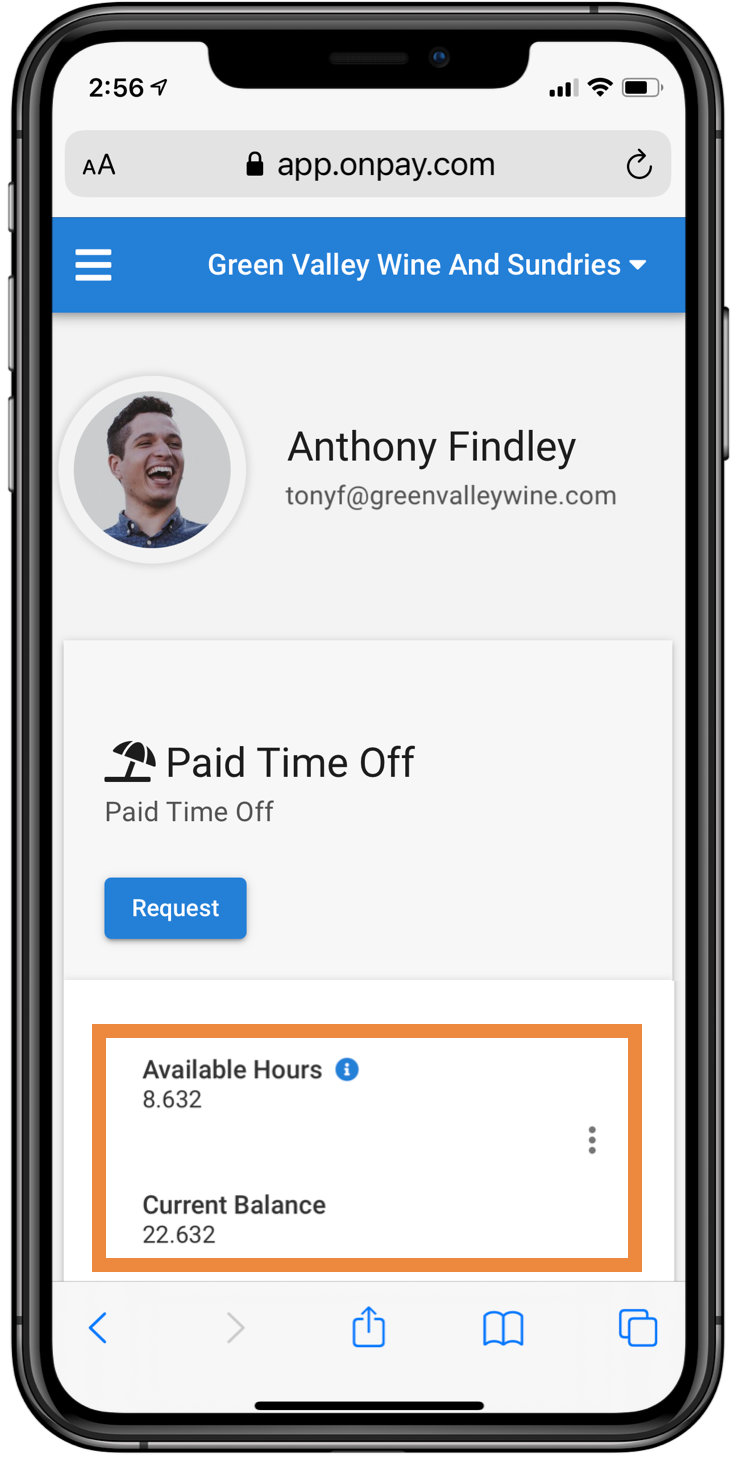The image depicts a full view of a smartphone, including its side buttons and edges, showcasing the screen content. The displayed screen is a webpage from the URL app.onpay.com. At the top of the page, there is a blue banner with the text "Green Valley Wine and Sundries," accompanied by a menu icon consisting of three horizontal lines on the left side, indicating additional options can be accessed.

Below the banner, there is a profile section featuring a profile picture of a smiling young man in a blue button-down shirt. His name, Anthony Findley, is displayed next to the picture along with his email address, tonyf@greenvalleywine.com.

Further down, an umbrella icon signifies the "Paid Time Off" section. Under this header is a blue "Request" button. Below this button, there is an area that details available paid time off hours, with the label "Available Hours" and an information icon next to it. The current balance is listed as "8.632" hours. Both the available hours and current balance are enclosed in a box highlighted in orange.